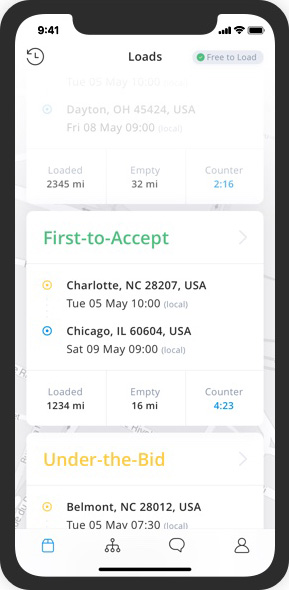This is a vertical rectangular image depicting a cell phone with a sleek black rim and rounded corners. The top-left corner of the screen displays the time as 9:41, alongside a refresh icon. Centered at the top, the word "Loads" is prominently displayed, and the top-right corner shows a full-strength cellular signal, a fully connected Wi-Fi signal, and a full battery icon.

Below this top section, the screen background transitions into a white or gray color. The next section shows text indicating a location and date: "Dayton, Ohio, ZIP code, Friday, May 8th at 9:00 AM." Underneath, statistical data is provided: "Loaded: 2345 MI, Empty: 32 MI, Counter: 216."

Further down, another box presents additional information: "First to Accept: Charlotte, North Carolina, Tuesday, May 5th at 10:00 AM; Chicago, Illinois, Saturday, May 9th at 9:00 AM." Additional stats follow: "Loaded: 1234 MI, Empty: 16 MI, Counter: 423."